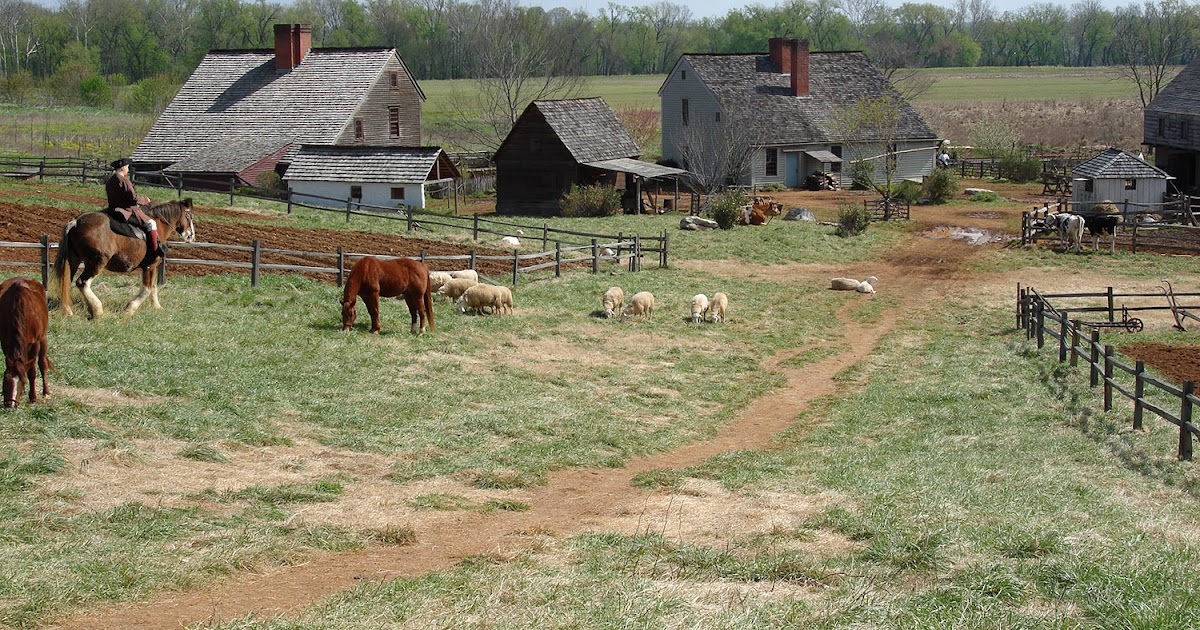The photograph captures a picturesque, slightly elevated view of a traditional farm scene, descending approximately 25-50 feet toward a cluster of rustic buildings. At the center is a two-story farmhouse with a sharply sloped roof and two distinctive red chimneys. To its left stands a dark brown shed, while further left is a larger, multi-story barn in medium brown with a single-story white section, possibly a stable.

The foreground features freshly plowed, fenced-off fields surrounded by wooden fences, suggesting recent preparation for planting crops. A dirt path winds through the grassy landscape, showing signs of frequent use by people and animals. On the left, a person rides a brown horse with white socks, accompanied by two smaller brown grazing horses. Numerous sheep roam freely, with some grazing and one lying down in the distance. Additional fenced pens, including a garden, are positioned to the right near the main farmhouse, alongside some other animals.

The scene is framed by a backdrop of trees, emphasizing the tranquility of the bright, sunny day on the farm, where various animals coexist in harmony amidst the lush green grass and pastoral surroundings.